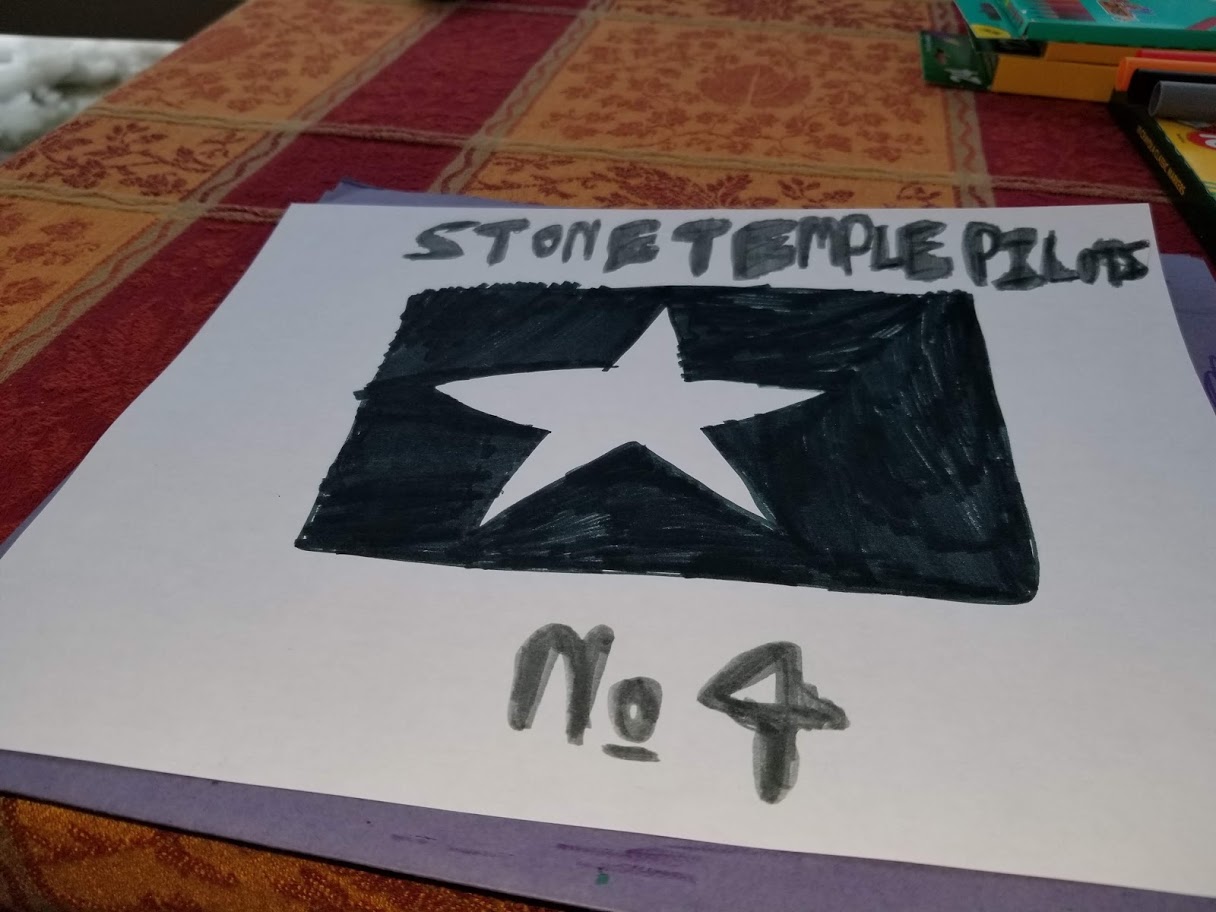A close-up photograph captures a handmade sign positioned on a table adorned with a vibrant floral-patterned tablecloth. The tablecloth features a design of maroon-colored flowers interspersed with a rich burgundy stripe running along either side. In the upper right corner of the image, various art supplies such as Crayola markers and colored pencils are visible. The centerpiece of the photograph is a white piece of A4 paper layered on top of a purple sheet. The sign, possibly created by a fan for a Stone Temple Pilots concert, is crafted with black marker and prominently displays the words "Stone Temple Pilots" at the top. Below the text is a black flag with a white star in the center, followed by the inscription "No. 4". The scene, viewed from a perspective suggesting personal involvement, has an amateur and authentic quality.